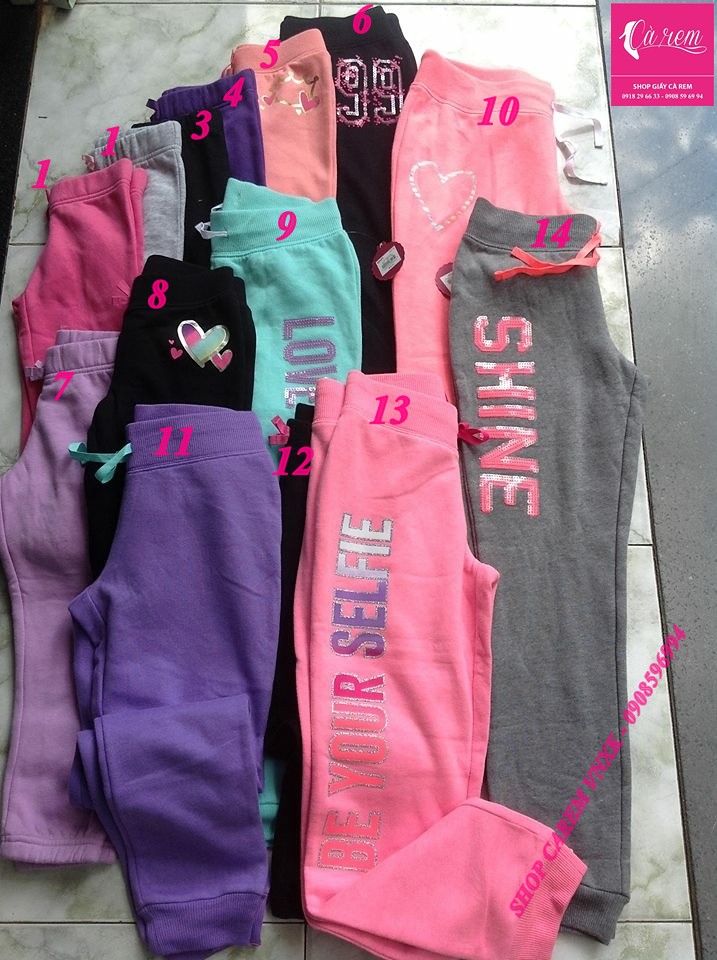This image features a meticulously arranged collection of 14 pairs of jogging pants displayed on a white marble floor with visible tile lines. These joggers are laid out in a staggered and slightly overlapping manner, revealing an array of colors including purple, pink, teal, gray, lavender, and peach. Each pair is numbered in pink, italicized font progressing from 1 to 14, though the number 2 is missing and the number 1 is repeated twice (1, 1, 3, 4, 5, 6, 7, 8, 9, 10, 11, 12, 13, 14).

The joggers each feature distinctive details: one gray pair has the word "SHINE" written in reflective pink letters, a pink pair displays "BE YOUR SELFIE" vertically along the leg, and a teal pair spells out "LOVE." Another black pair (number 6 in the grid) has the number "99" at the top. The pants are designed with elastic waistbands and tapered ankles, typical of standard joggers.

In the top right corner, there is a pink square containing the logo "SHOP CAREM" accompanied by a phone number, suggesting this image originates from an online store's product catalog. This detailed presentation allows potential buyers to easily identify and select their preferred pair based on the corresponding number.